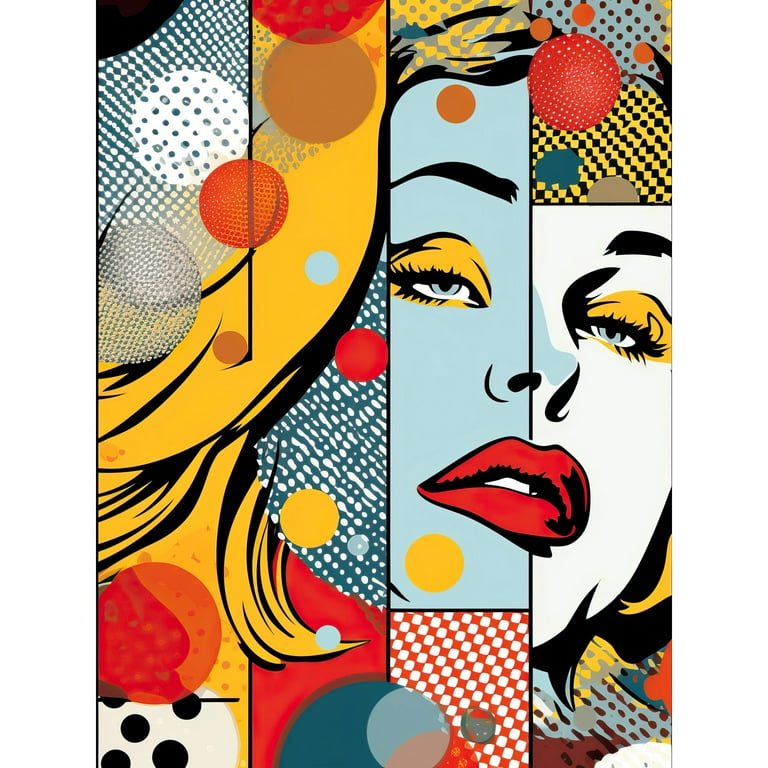The image is a vibrant pop art piece showcasing a woman's face composed of distinct, separate boards that are meticulously divided by thin black lines. The woman's visage is striking, featuring blonde hair and bold red lipstick. Her face is intriguingly split, with one side rendered in stark white and the other in a contrasting teal shadow, highlighting her sharp pointy nose. She wears yellow eye shadow, adding to the vivid color scheme. The background and sections of her face include a variety of patterns and textures, such as plaid and polka dots, creating a dynamic collage effect. Scattered throughout the piece are numerous colorful spheres, enhancing the complexity and richness of the artwork. The overall composition blends retro styles with modern digital art techniques, resulting in a visually compelling and multifaceted portrait.